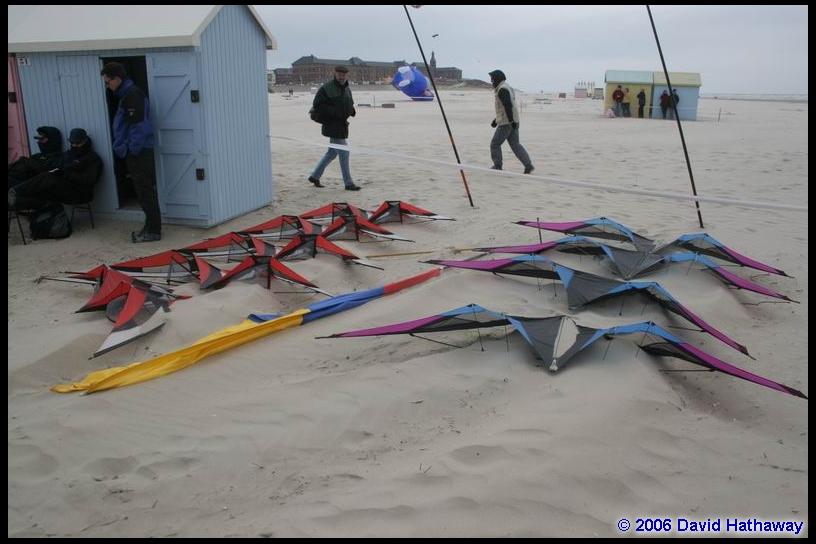The scene is set on a sandy beach where various kites are lined up meticulously. On the right side, there are four kites in a row, each with a gradient design spanning from black in the middle to blue, then purple, and ending in black points. Just to the left of them lies a flag, stretched out thin like a stick, featuring sections of yellow, blue, and red. Adjacent to these kites, moving left, another row of kites appears, predominantly red with black and white strips. A white rope barrier with black sticks is positioned in front of the kites. Behind this barrier, a man in a light tan vest with long black sleeves walks leftward, while another man in a dark green jacket and blue jeans walks in the opposite direction.

In the upper left-hand corner, there's a blue and white storage shed with an open door. A man, wearing a blue jacket over his head, stands in the doorway. Two shadowy figures lean against the shed. Further in the background on the right, two buildings — one blue, the other yellow — stand side by side, with five people gathered in front. An additional, larger building can be seen in the distant background. The lower right corner features blue text with a copyright symbol, marked "© 2006, David Hathaway."